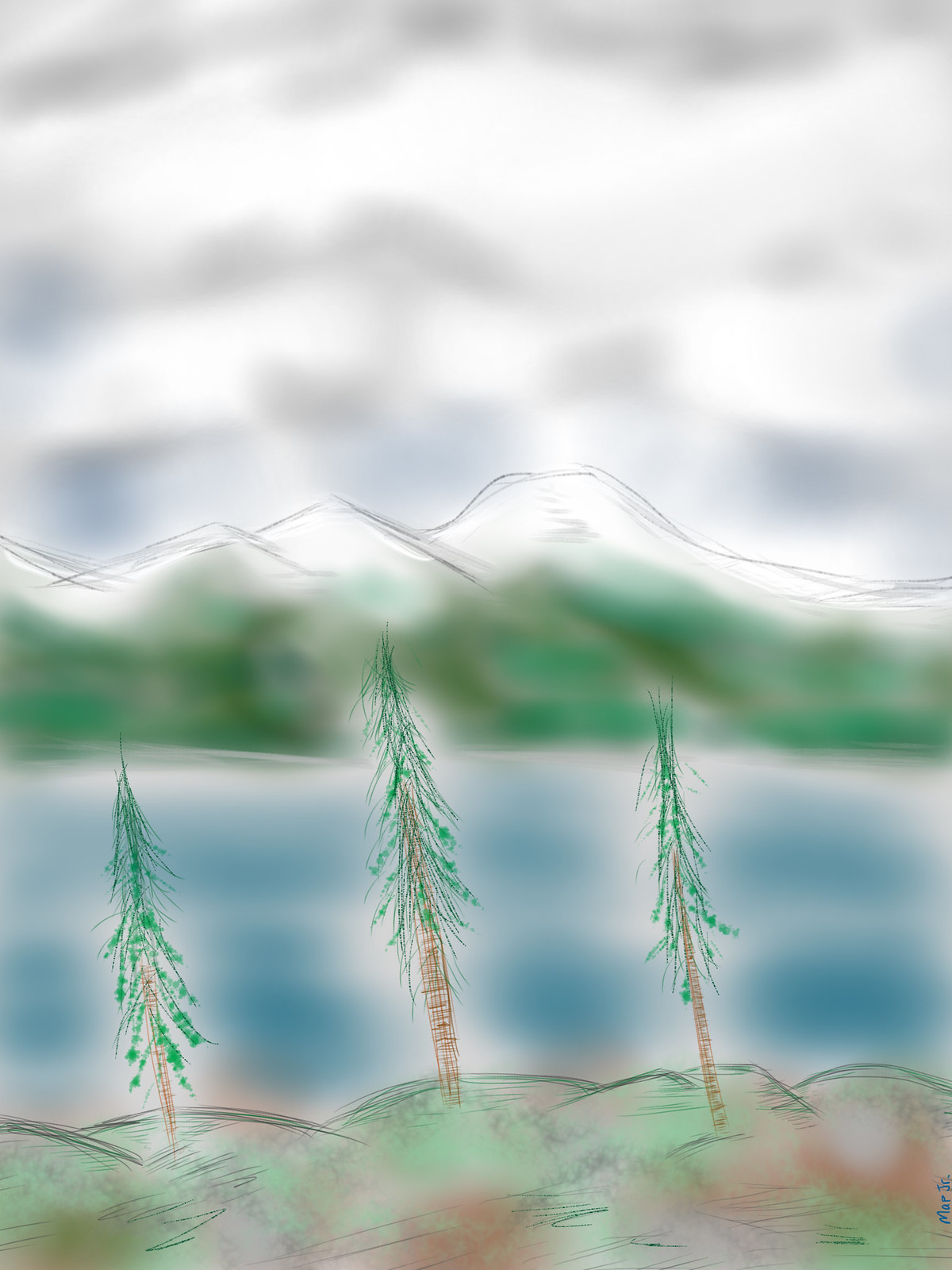This artwork beautifully captures a serene landscape scene. The background is comprised of a vivid sky, adorned with a mix of white and gray clouds that add depth to the piece. Beneath the sky, majestic mountains, appearing snow-capped and white, tower over the horizon. The midsection of the painting features an expansive area of green, somewhat blurred to imply lush vegetation on the mountain slopes. Below the green terrain, a tranquil body of water is depicted in shades of blue, interspersed with white lines that suggest the play of light on the water’s surface. In the foreground, a stretch of brown soil adds an earthy element to the composition, with textured bumps enhancing the realism of the terrain. Three prominent trees stand tall amidst the dirt, their brown trunks rising from the ground and branching out into gray leaves that lend an ethereal quality to the foliage.